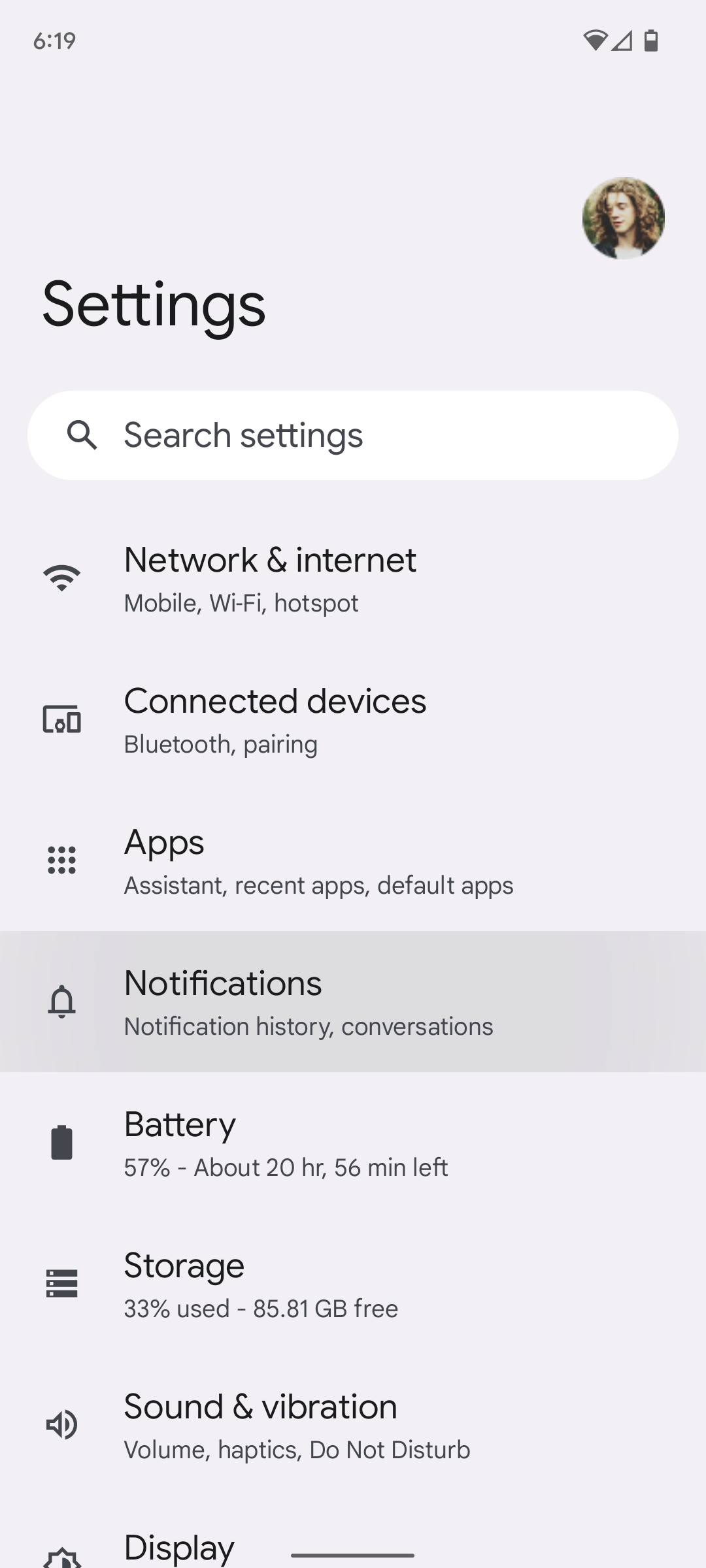The image is a screenshot taken from an Android device, as evident from the user interface elements. In the top left corner, there is a number "619". On the top right corner, there is a Wi-Fi icon, followed by a signal icon showing no reception, and then a half-full battery icon. 

Below these icons, there is a circular profile picture of a person, who appears to be a white male with blondish hair, looking slightly to the right. The clarity of the image is not high, making detailed facial features hard to discern.

Directly under the profile picture is the word "Settings," followed by a large, white, oval-shaped search bar labeled "Search settings." Below this, various menu options are listed in a sequence:

1. **Network and Internet:** Includes "Mobile, Wi-Fi, Hotspot"
2. **Connected devices:** Indicates "Bluetooth pairing"
3. **Apps:** Lists "Assistant, recent apps, default apps"
4. **Notifications:** This section is highlighted in gray and includes "Notification history, conversations"
5. **Battery**
6. **Storage**
7. **Sound and Vibration**
8. **Display:** This section is partially cut off.

Each menu item is accompanied by a corresponding icon on the left-hand side.